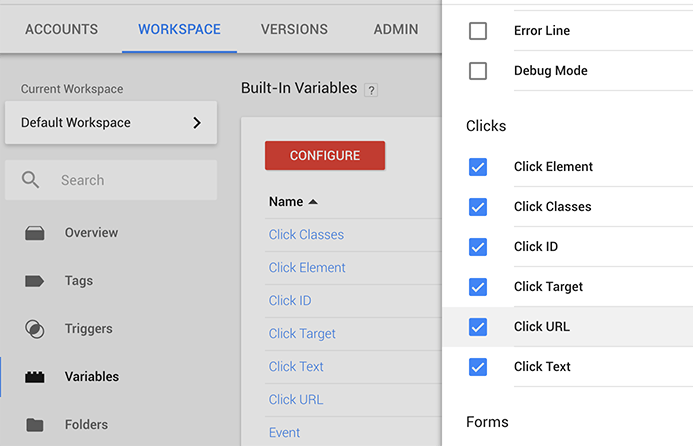The image depicts a screenshot of a Google Workspace application, probably Google Tag Manager, given its workspace-related functionalities. At the top left corner, the menu includes options such as Accounts, Workspace Versions, Admin, with the Workspace tab highlighted in blue, indicating it is currently selected. Below this menu, various workspace-related terms are present.  

A central search bar is visible, accompanied by a configuration button used for creating elements. Beneath these are a series of options for creating and monitoring items like Click Classes, Click Element, Click ID, Click Target, Click Text, Click URL, and event. Each of these creation options can be checked off, and in the image, all are checked off except for Airline and Debug Mode, which remain unchecked.

On the left side panel within the screenshot, it is evident that the user is in the "Default Workspace," as indicated at the top. Underneath the search bar, the menu options displayed are Overview, Tags, Triggers, Variables, and Folders. The Variables tab is actively selected, distinguished by its black color, contrasting with the gray of the other options.